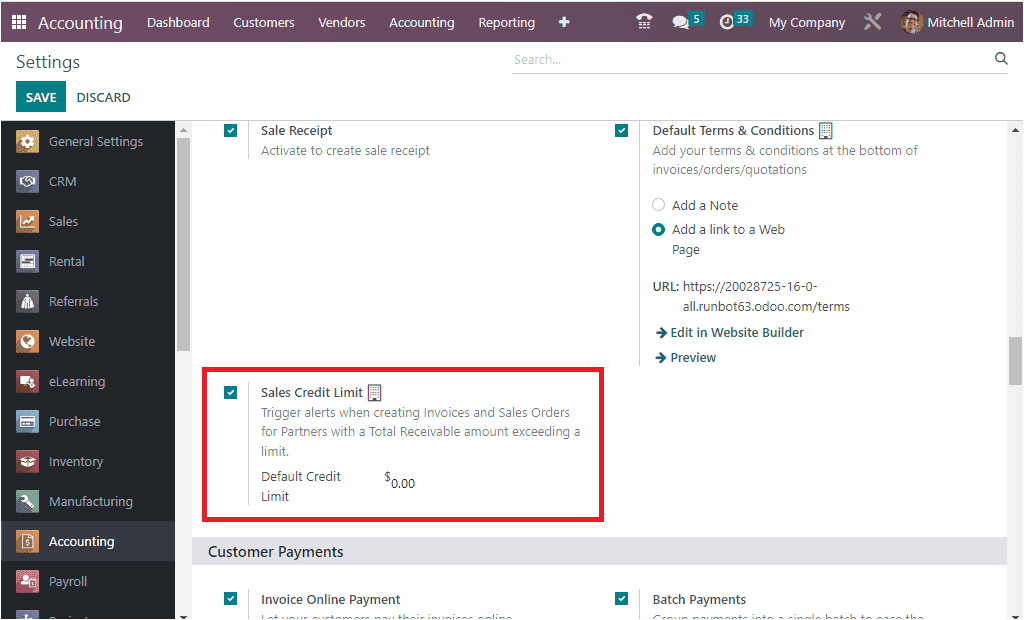**Detailed Screenshot Description:**

The image is a screenshot of a web browser interface specifically tailored for accounting purposes. The browser header is wine-colored, featuring the word "Accounting" on the top left. Aligned on the same row are menu tabs: "Dashboard," "Customers," "Vendors," "Accounting," and "Report." Additionally, there are several icons: a plus sign for adding new entries, a talk bubble icon with a notification badge showing the number 5, a clock icon with the number 33 indicating pending tasks or alerts, and at the far right, the username "Mitchell Admin".

On the left sidebar, which has a black background, there is a scroll bar indicating more options can be viewed by scrolling. The sidebar section under "Settings" includes a "Steal Save" button and a "Discard" button. General categories listed in the sidebar include: "General Settings," "CRM," "Sales," and "Rental," among others, each accompanied by a corresponding icon.

The main body of the webpage has a white background and is divided into two sections. The upper section is headed "Sales Receipt." The lower section, highlighted with a red border, details settings related to "Sales Credit Limit," including a trigger alert for exceeding receivable limits when creating invoices and sales orders for partners. Next to this, there is a green checkmark, indicating these settings are enabled. Also located here are options for "Default Terms and Conditions," with two selectable choices: "Add a Note" and "Add a Link to a Webpage," with the latter currently selected. Additional links for "Edit in Website Builder" and "Preview" are also present.